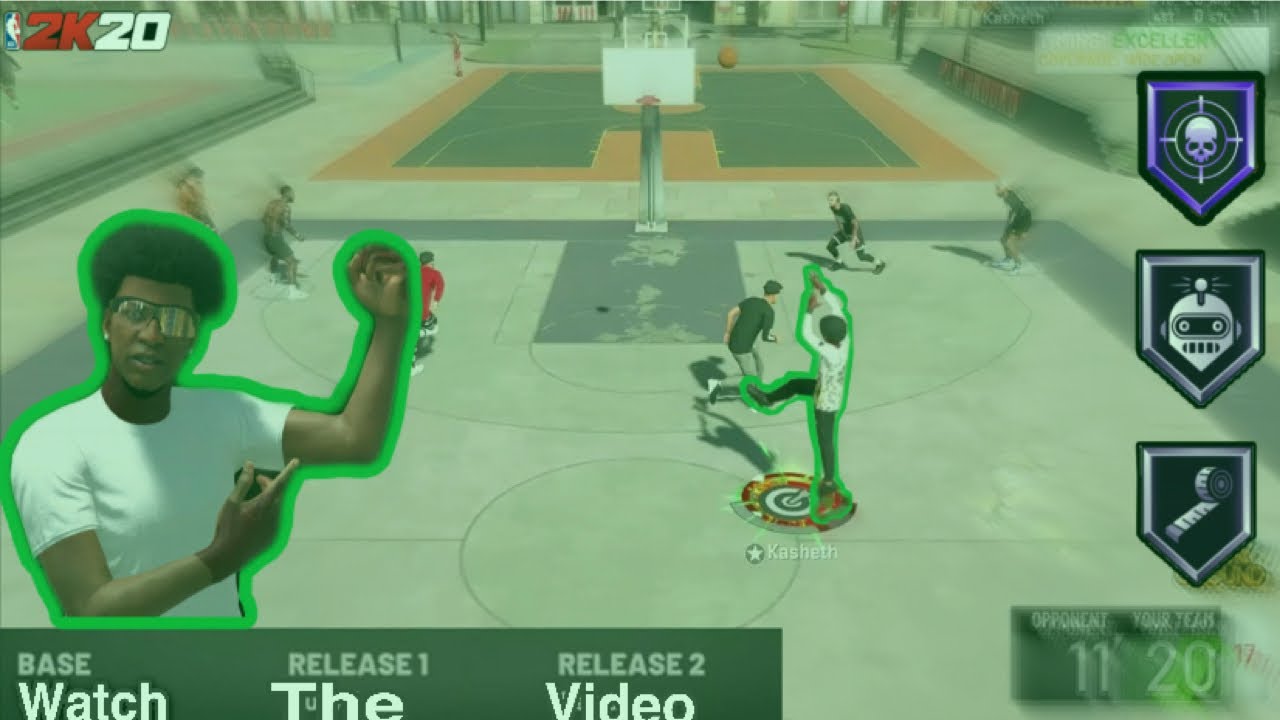In this vibrant and action-packed NBA 2K20 gameplay image, an African-American player, identified as "Kashef," is captured mid-shot against a realistic green basketball court backdrop. Kashef, dressed in a white shirt and black pants, is outlined in green and highlighted with his name in white and a white star on a grey background beneath him. Taking center stage, Kashef is in the midst of an intense play, aiming for the basket. His athletic prowess is emphasized by his pose; pointing to the muscle in his left arm, wearing reflective sunglasses, and sporting an Afro, he exudes confidence and power. The text "base, release, and release two" is prominently displayed, guiding players through gameplay mechanics, along with a prompt to "watch the video" at the bottom of the screen.

In the scoreboard, Kashef’s team leads with a score of 20, against the opponent's 11. Overlay icons add layers of depth to the scene. A prominent icon features a skull centered inside crosshairs, shielded by a purple and black design. Below it, a robot encased in a silver and black shield is visible, alongside a measuring tape icon similarly framed. Six additional players are active on the court, adding to the dynamic and competitive atmosphere. The shadow and bullseye surrounding Kashef enhance his dramatic presence on the court.